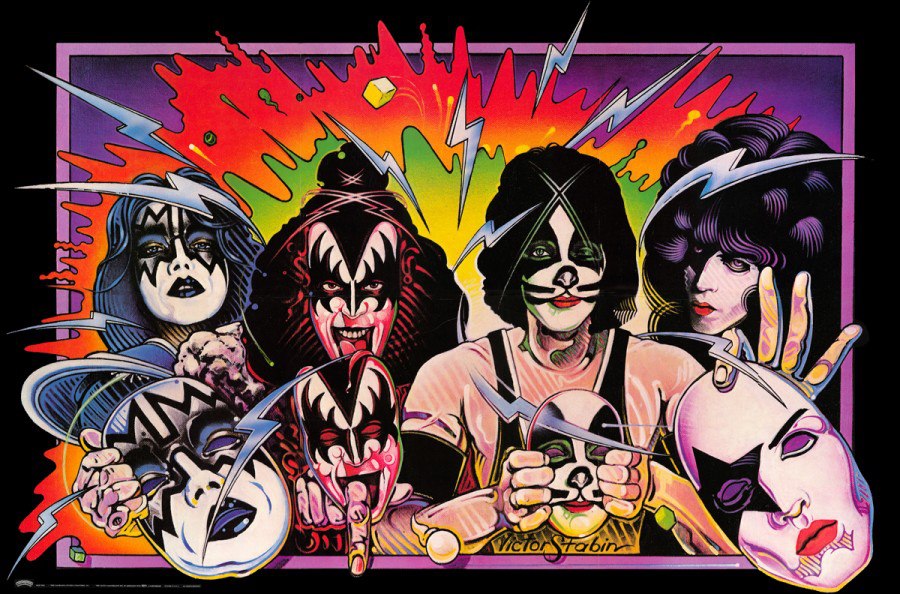This vibrant and detailed artist's portrayal of the iconic band Kiss features all four members front and center, each showcasing their signature makeup and black hair. The composition is horizontally rectangular, with a bold black outline framing the image, followed by a pink border and a purple inner frame. The central background behind the band members transitions through splashes of vivid yellow, green, and orange colors, mimicking a paint-splatter effect, while darker purple fills the outer background.

Each band member holds a ceramic mask that mirrors their own painted faces. Starting from the left, the first member dons black and blue star-themed makeup with blue lips and highlights in their hair. The second member, recognizable as Gene Simmons, has a striking bat-wing design around his eyes, complete with a wide-open mouth revealing a tongue, partially obscured. The third member presents a cat-like appearance with green eyeshadow, black 'whiskers' extending from the nose, and red lips; he's dressed in a short sleeve pink shirt over a black outfit. Finally, the fourth on the far right displays a mask with black star makeup on the left eye and red lips.

Lightning bolts and zigzag silver lines emanate from above their heads, adding dynamic energy to the scene. The poster is signed at the bottom by the artist, Victor Stabin, solidifying its authenticity. The intricate decorative details, each band member's unique persona, and the explosion of colors capture the electrifying presence of Kiss in this captivating art piece.